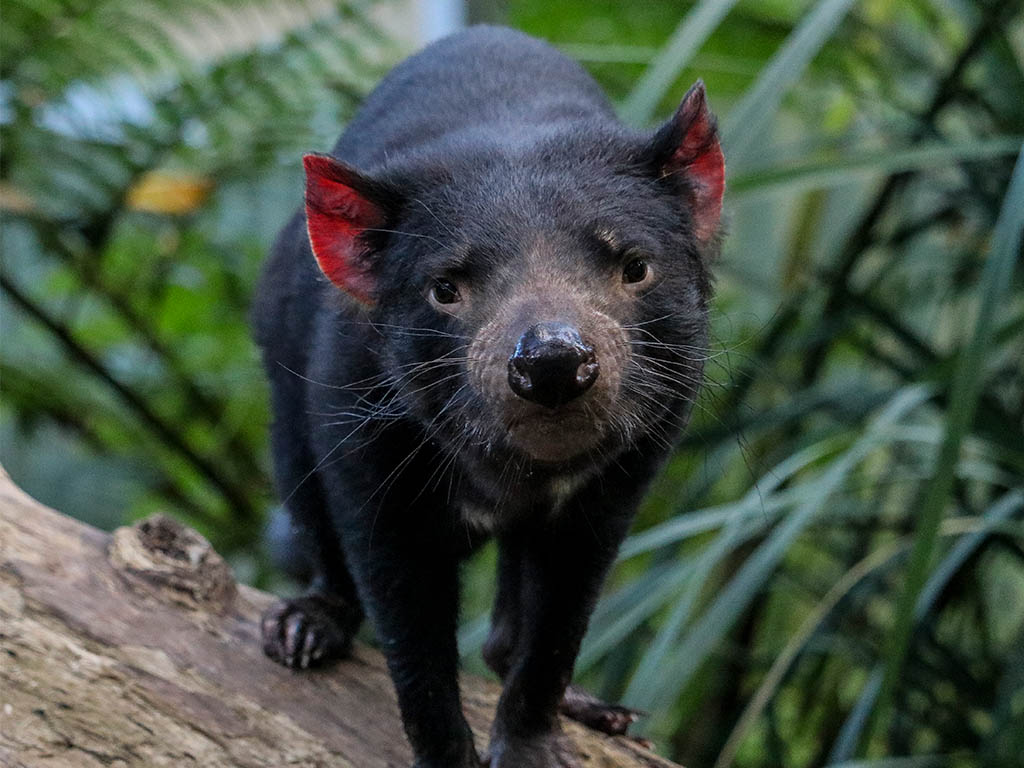This close-up image captures a Tasmanian devil standing on a fallen log amidst a jungle-like setting. The Tasmanian devil is small, almost cat-sized, with black wiry fur covering its body. Its face features black beady eyes that stare directly at the camera, a large dark black nose, and prominent whiskers. The snout is partly light-colored, transitioning to a deep black at the tip. The animal has pointy, triangular ears that are pinkish-red on the inside and covered in black fur. Its sharp claws are visible on both the hind and forefeet, gripping the log. The background is a blur of lush greenery, including shrubs and possibly palm trees, further emphasizing the vivid focus on the Tasmanian devil and its perch.